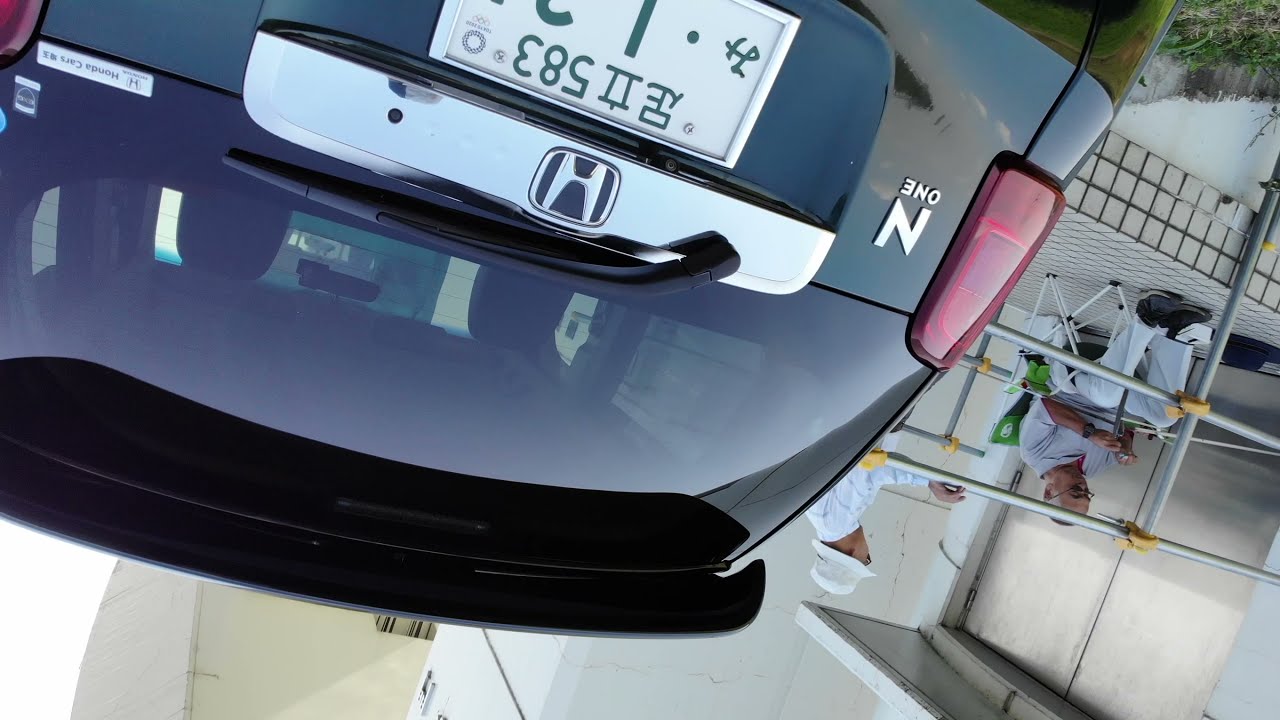This image, taken upside down, prominently features the back of a black SUV, likely a Honda, as indicated by the "H" symbol in the middle of the vehicle. The license plate, positioned at the top of the picture due to the orientation, contains characters in a foreign language along with the numbers "583." The SUV has a tinted back window and a visor meant to provide shade. To the left of the taillight, there is a marking that reads "N1." 

In the center right of the image, there are two individuals. One person is seated in a chair, wearing glasses, black shoes, and appears to have a shaved head. They are looking downward, possibly at something on their lap, and are sitting next to a white building. The second person, standing close to the car, is dressed in white, including a white cap. They seem to be reaching for or serving something.

The setting seems to be an outdoor patio with a stone or tiled floor, surrounded by metal-looking bars. The image shows a reflection of the sky in the car's window, hinting that the photo was taken in daylight. The overall colors in the scene include black, white, gray, tan, green, red, and blue.